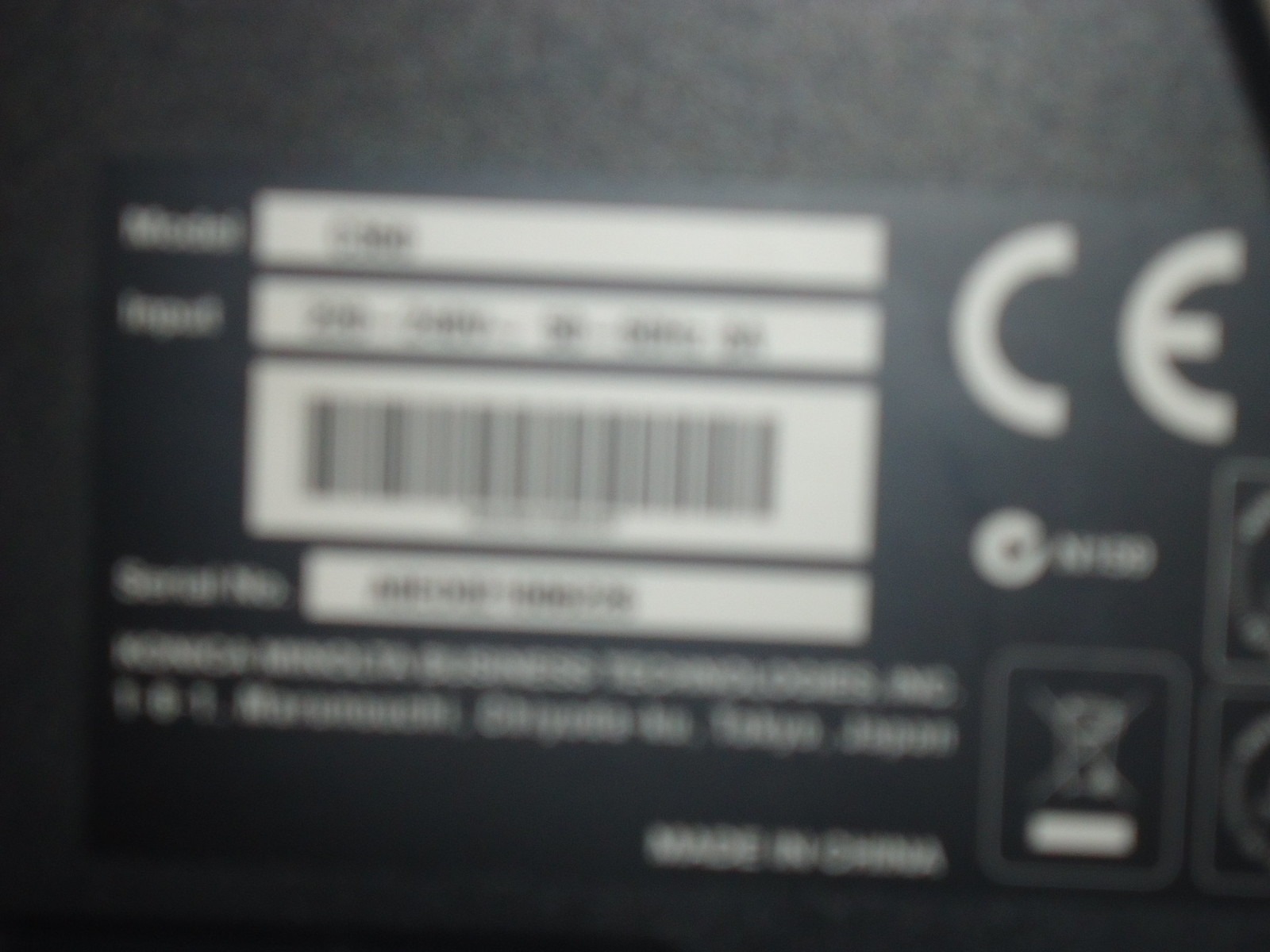The photograph depicts a blurry and dimly lit image of a barcode label. Situated towards the top center is a light source that partially illuminates the scene. 

At the top left of the image, the word "model" is visible in white letters. Adjacent to it on the right is a rectangular white box containing indistinguishable black text due to the blurriness. Below this, there is more white text on the left and another white box with black writing on the right, also unreadable. 

Directly beneath this is a larger white rectangular box of the same width, containing the barcode itself. Underneath the barcode box is another rectangular box with further indistinguishable black lettering. 

The bottom section features additional white text. To the right of the stacked rectangular boxes, large white letters "C" and "E" can be seen. Below these letters, there is a symbol of a crossed-out circle, indicating that the item should not be disposed of in regular waste bins. 

Overall, the poor focus and lighting make the specific details difficult to discern, but the general layout and elements are identifiable.